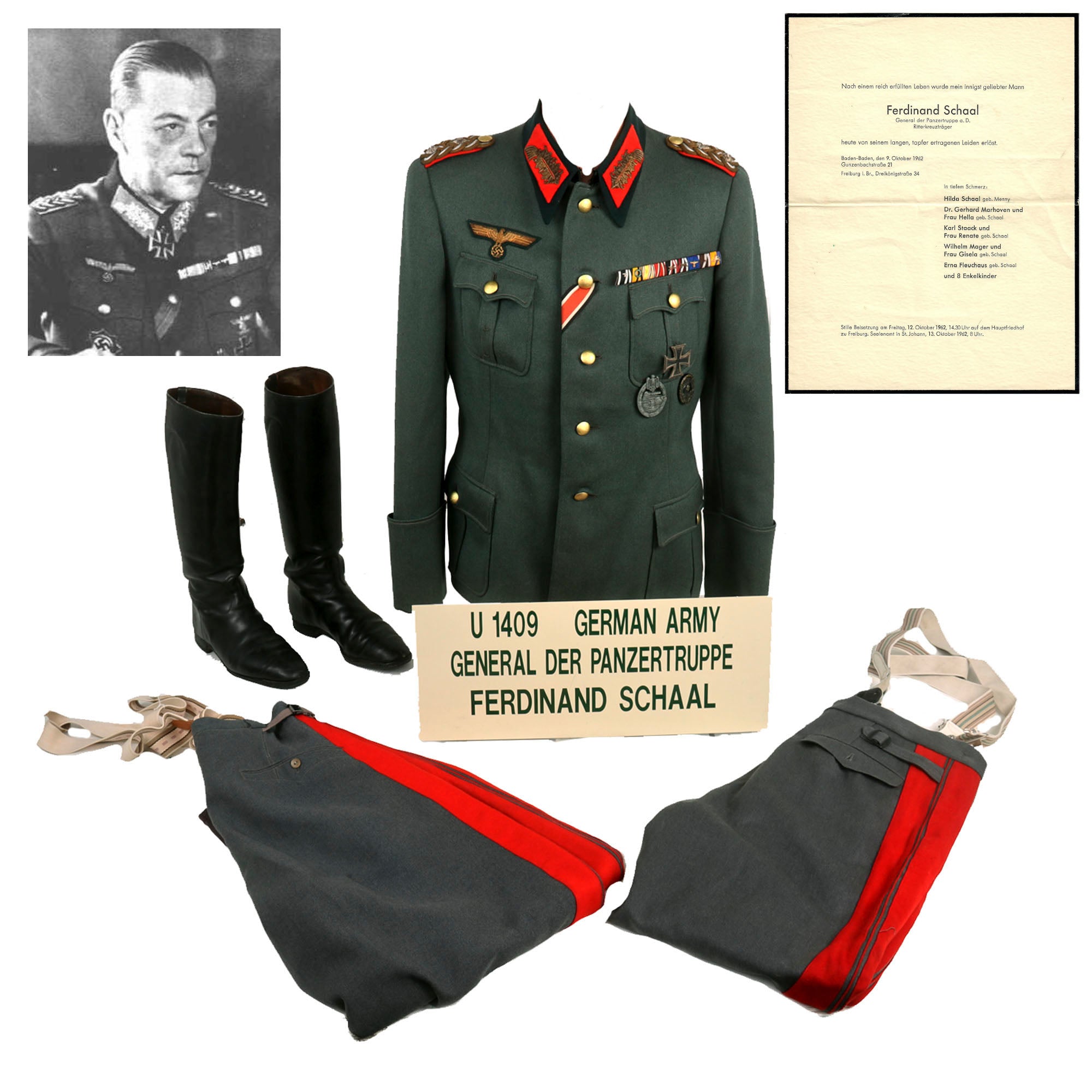The image presents a detailed display typically found in a history museum, showcasing artifacts related to a German military veteran named General der Panzertruppe Ferdinand Schall. At the center, a dark olive-green or dark emerald-green military uniform, resembling a long-sleeved jacket or blazer, prominently stands out. The jacket features red lapels adorned with gold feathers and gold buttons down the middle. Among these buttons, a red, gold, and black stripe is noticeable under the second button. Medals, including a bronze cross, a silver medal, and possibly a tarnished bronze or black medal, are arrayed on the right side of the jacket. 

Beneath the jacket is a beige sign with green lettering stating "U-1409, German Army, General der Panzertruppe Ferdinand Schall." Below the jacket, gray pants with red stripes are visible, and to the left, tall black boots are positioned. 

In the upper left of the montage, there is a black-and-white photograph of a man, likely Ferdinand Schall, dressed in a similar uniform. On the top right, a beige document displays Ferdinand's name and additional smaller, less legible text, resembling a letter or commendation. Together, these elements create a comprehensive and detailed portrayal of the military service and accolades of General Ferdinand Schall.